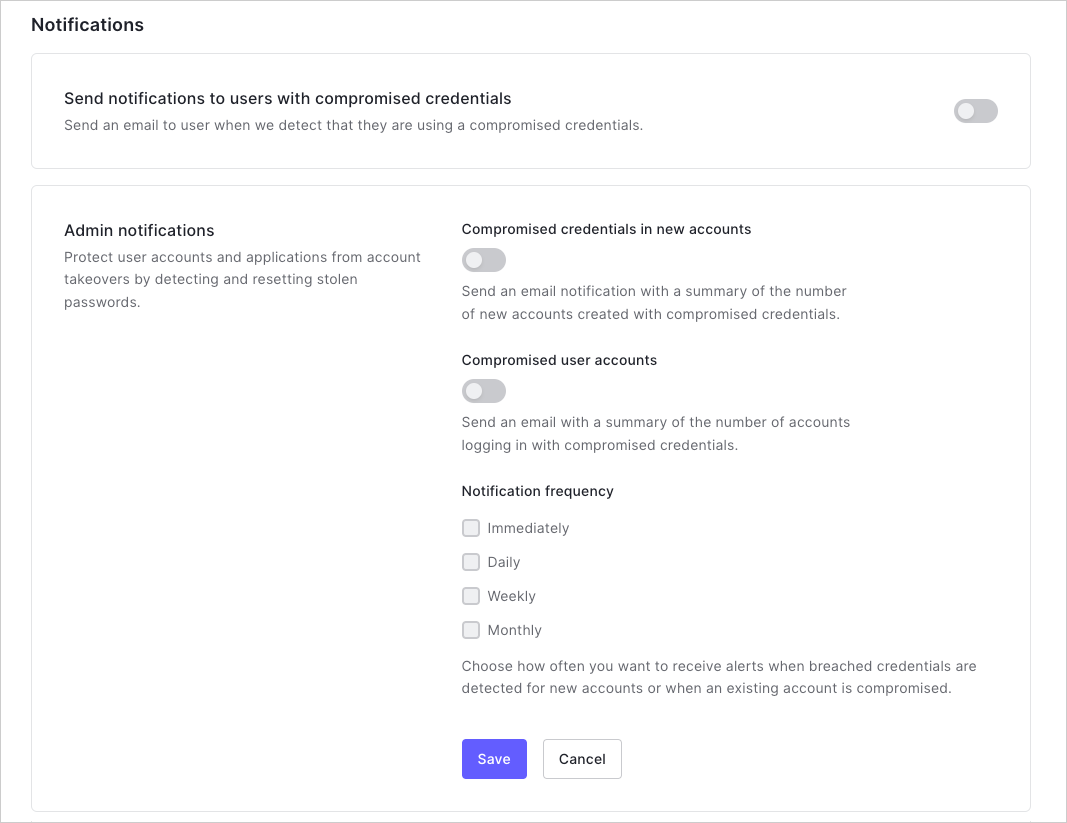This image is a detailed screenshot of a notification settings interface related to compromised credentials. 

At the top left corner, the header "Notifications" is displayed in black text. Below this header, the section titled "Send Notifications to Users with Compromised Credentials" outlines various options:
1. "Send an Email to User When We Detect They Are Using a Compromised Credential."
2. "Admin Notifications" on the left, with "Compromised Credentials and New Accounts" on the right. These options encompass:
   - "Send an Email Notification with a Summary of the Number of New Accounts Created with Compromised Credentials."
   - "Send an Email with a Summary of the Number of Accounts Logged in with Compromised Credentials."

Further down, the "Notification Frequency" section offers four vertical options for setting how often notifications are received: 
- Immediately,
- Daily,
- Weekly,
- Monthly.

The description below these options states: "Choose How Often You Want to Receive Alerts When Breached Credentials are Detected for New Accounts or When an Existing Account is Compromised."

Towards the bottom, there are two buttons:
- A blue "Save" button on the left.
- A "Cancel" button with black text and a white background on the right.

The entire interface is set against a white background.